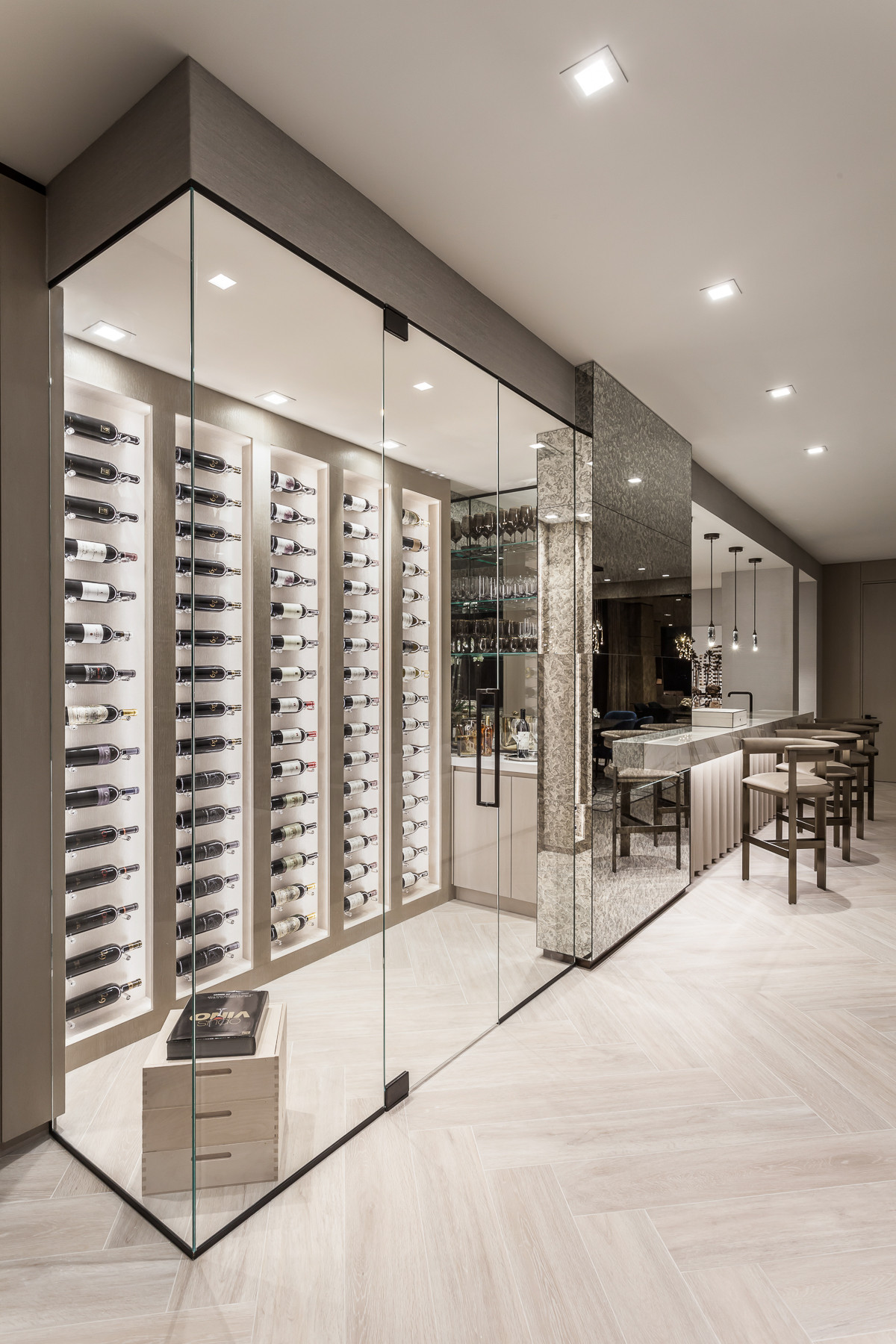This vertically aligned rectangular picture showcases a meticulously clean and well-organized modern wine room. Dominating the left side is a large shelf enclosed behind glass doors, featuring five rows of wine bottles arranged horizontally, almost reaching from floor to ceiling. The bottles have varied labels, some solid black and others with white labels. On the right side, a counter with a gray marbled countertop is accompanied by several high-back cushioned chairs. Above this bar area, three pendant lights hang from the ceiling, casting light over the counter. The white ceiling features additional square-shaped ceiling lights emitting a bright light. The lower right section of the image highlights a distinctive zigzag pattern on the tile flooring, blending brown and light gray hues. The overall color palette of the room includes shades of silver, gray, light gray, black, off-white, and tan. In the bottom corner, a wooden box with a book on top can be seen through the glass. This indoor setting emphasizes a sophisticated and upscale atmosphere, indicative of a dedicated space for wine storage and appreciation.